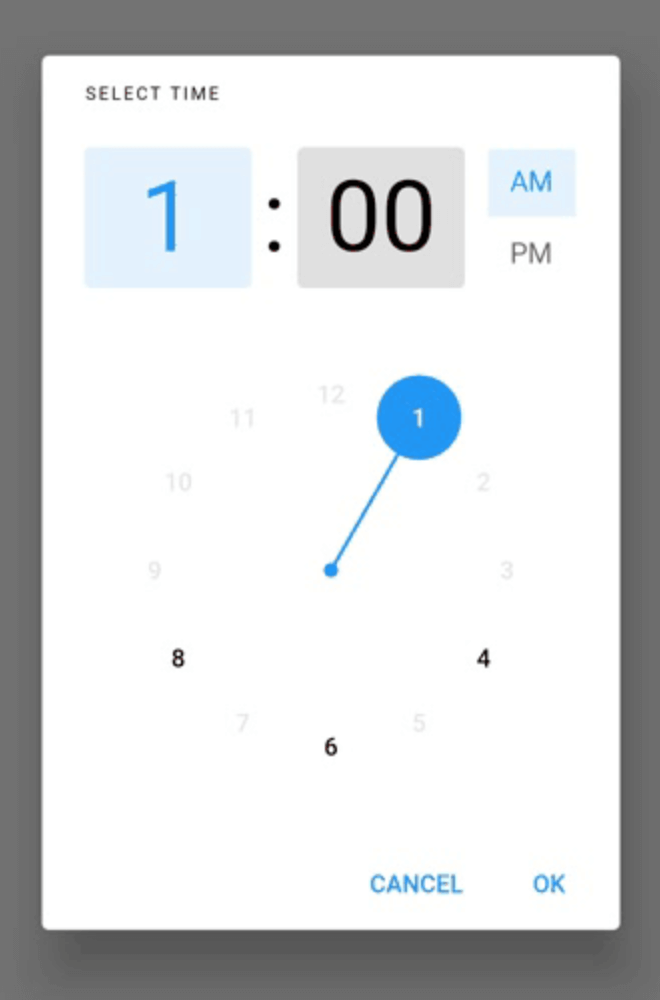The image depicts a digital clock interface for setting the time, likely on a smartphone or tablet. The background is a vertical gray rectangle with a white vertical rectangle layered on top. In the upper left corner, the text "SELECT TIME" is displayed in gray capital letters. 

Below this text is a series of elements to set the hours and minutes. On the left side, there is a blue square with a darker blue digit "1" inside. To its right, a colon separates it from another square. This square is gray with black digits showing "00". Next to the minute setting is a vertical selection labeled with "AM" and "PM". The "AM" option is highlighted in a smaller blue square, while "PM" is in gray.

Below these settings is a circular clock face. Most of the numbers on the clock are light gray, almost blending into the white background, except for the numbers 4, 6, and 8, which are bold black, and the number 1, which is white with a blue circle around it. A blue line extends from the number 1 to the center of the clock, which has a small blue circle.

In the bottom right corner of the interface, there are two buttons labeled "CANCEL" and "OK" in blue. The overall design suggests the interface is intended for setting the time, possibly within a mobile app. The detailed layout hints at a user-friendly way to manually enter and confirm the desired time.